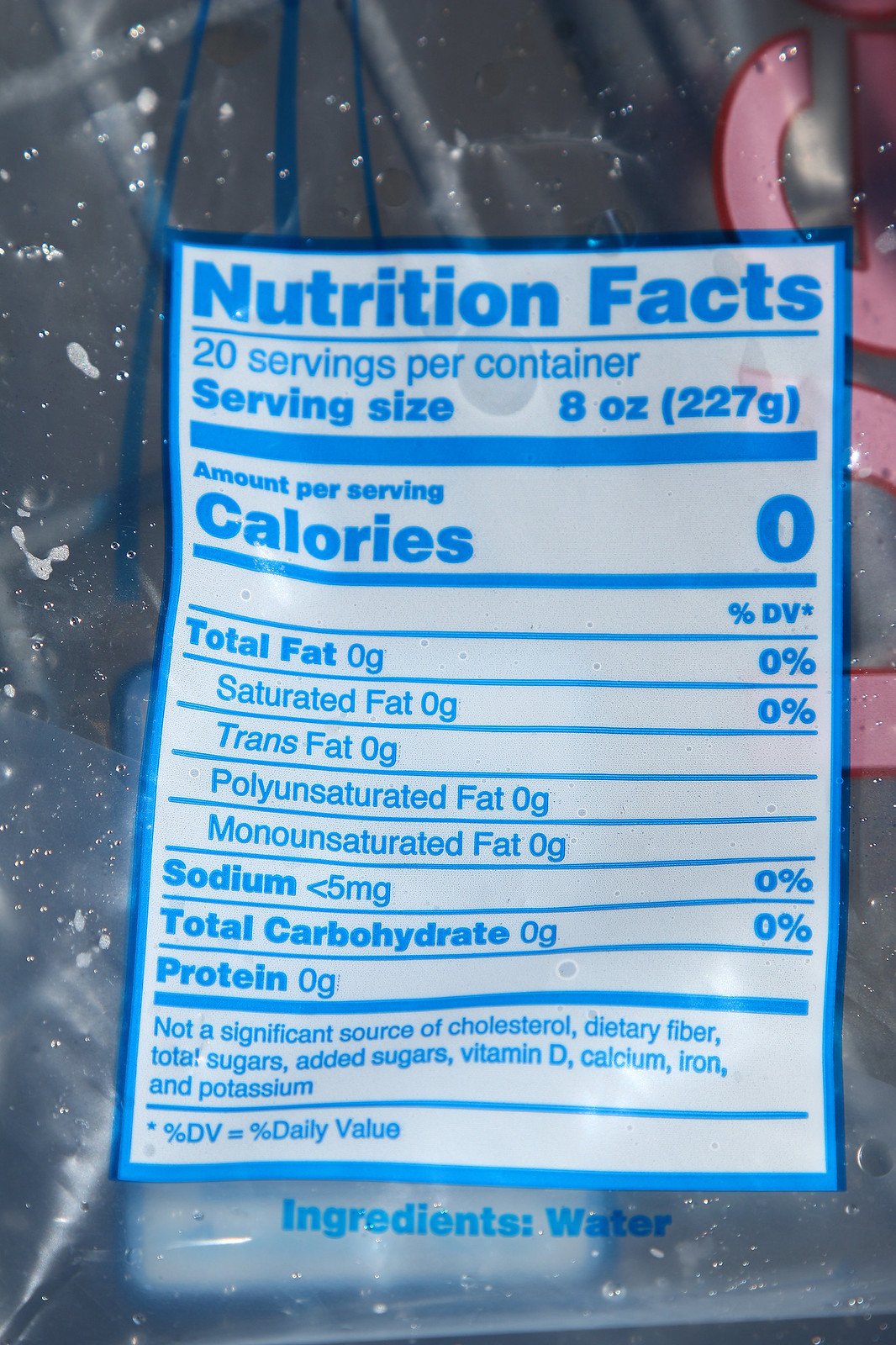This image features the Nutrition Facts label of a product which appears to be an ice bag. The label is printed in light blue font and indicates that the bag contains 20 servings, with each serving size being 8 ounces. Given that all nutritional values, including total fat, trans fat, polyunsaturated fat, sodium, carbohydrates, and protein, are marked as zero, it is clear that the product is essentially water. This assumption is further supported by the sole ingredient listed: water. The image does not provide any additional details about the bag itself, aside from a faint, unidentifiable logo situated behind the Nutrition Facts label. Overall, the image focuses exclusively on the nutritional information of what is presumably a bag of ice.